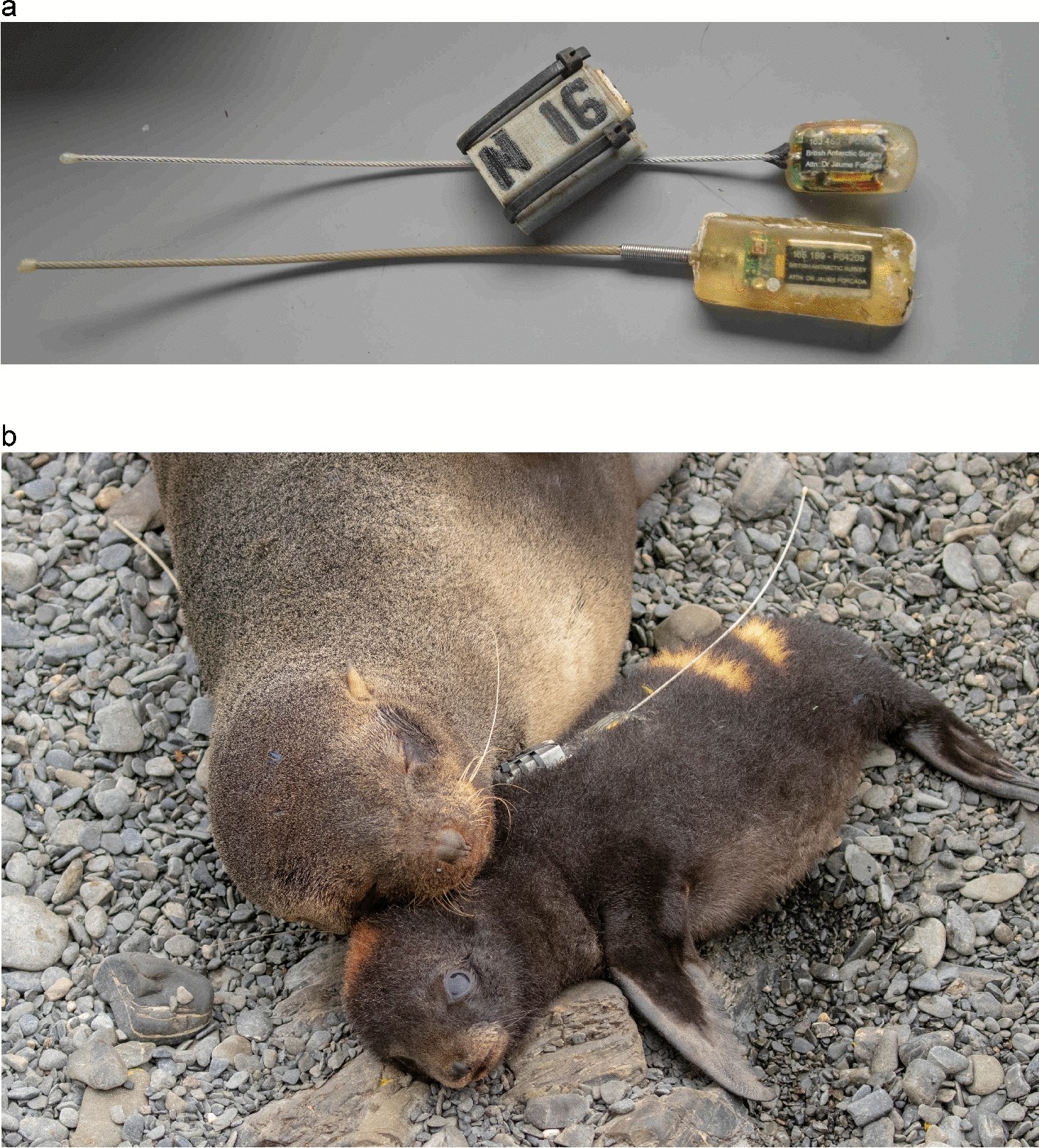The composite image consists of a top and bottom section. The top image displays two sets of tracking devices on a gray background. These devices appear to be braided strings, each attached to a plastic molding with labels. One device prominently features a metal slab marked with "IN16" in black marker. The bottom image depicts two animals, likely seals or sea otters, resting on a bed of small rocks. One of the animals, a juvenile or baby seal with its eyes open, has one of the tracking devices attached to its body. The larger animal, possibly the mother seal, is positioned with its head resting gently on the smaller one. This setup suggests that the tracking devices are being used to monitor the animals, but their presence and the positioning of the devices raise concerns about the well-being of the seals.